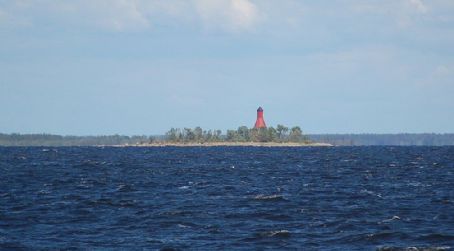This color photograph captures a vibrant coastal scene featuring a choppy expanse of dark blue water with distinct white caps. The horizon is flat and lined with distant land, densely populated by trees. In the foreground, there is an island with a brown coastline and lush green foliage. Prominently situated on this island is a tall, red tower that appears to be a lighthouse, crowned with a black top reminiscent of a factory stack. The sky above is mostly a light blue, adorned with wispy clouds at its upper reaches, and the sun remains hidden, indicating it's the middle of the day. The combination of the dynamic waves and the striking lighthouse against the natural backdrop creates a picturesque and vivid scene.